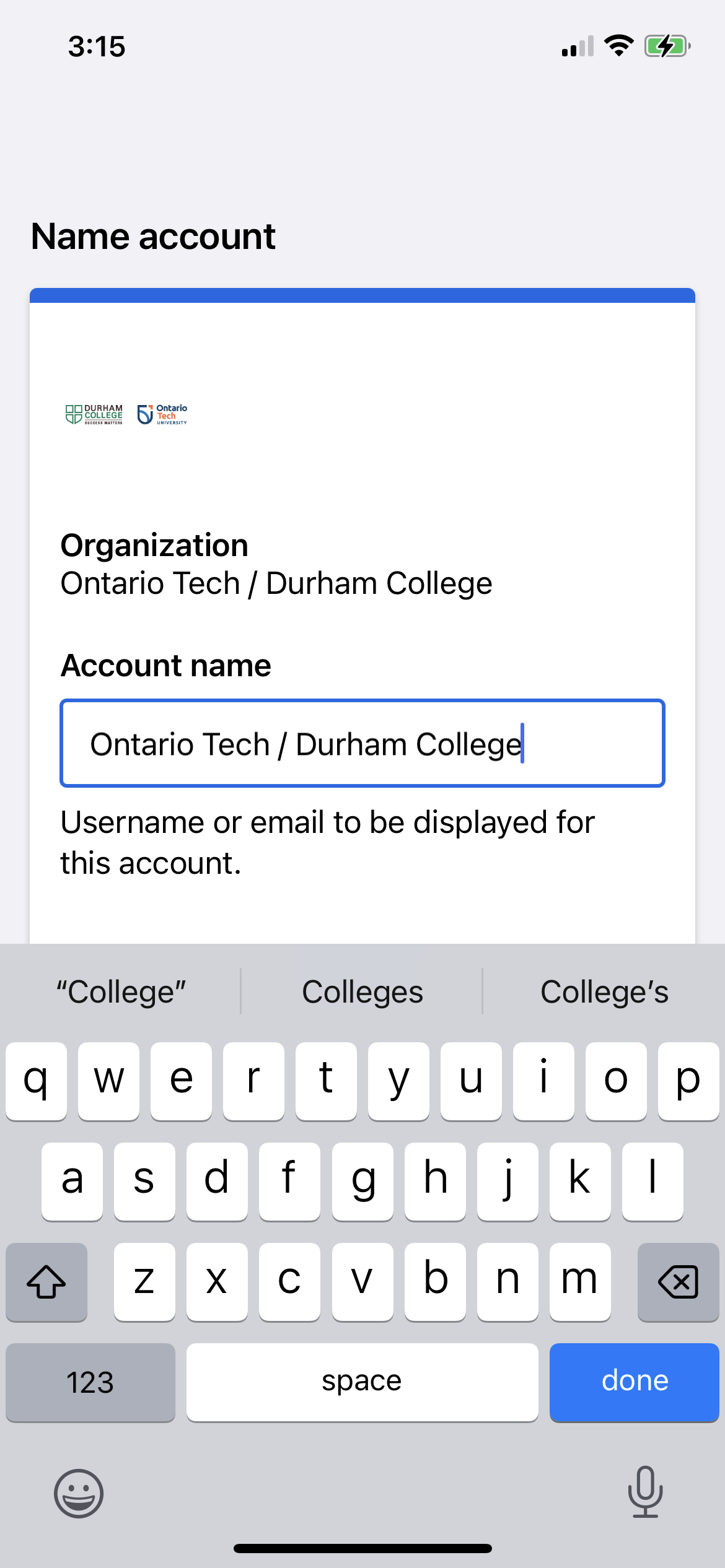A detailed, cleaned-up caption for the given image might be:

"This screenshot, taken on an iPhone at 3:15 PM, shows a user logged into their account associated with Ontario Tech Durham College. Notable details include two bars of cellular signal and a Wi-Fi connection, with the phone battery nearly fully charged and currently being charged. The visible interface includes fields labeled 'Organization Name: Ontario Tech Durham College' and 'Account Name: Ontario Tech Durham College', suggesting a possible error where the same name is repeated. The user had accessed their keyboard, but aside from a little blue line under the 'Account Name' field, there's minimal additional information displayed. This scene might depict a college student managing their academic account or seeking specific information related to their institution."